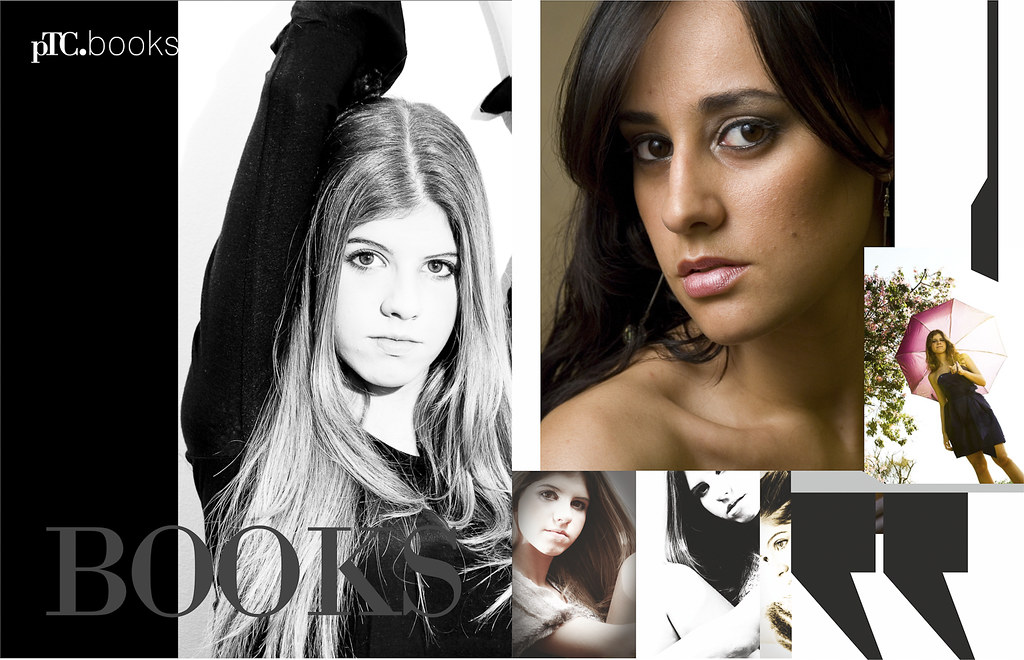The image is a collage of multiple fashion photographs, each depicting a close-up of a woman, possibly a model, with long dark hair. The overlaid photographs vary in style, with some in vibrant color and others in black and white. In the bottom left-hand corner, gray text reads "BOOKS," and a vertical black strip on the left side contains the white text "PTC.BOOKS." Within this strip, a black and white photo of a woman with her right arm raised above her head captures her staring directly into the camera. Further to the right, a colorful photograph features a woman holding a pink umbrella, set against a backdrop of trees and bushes, with smaller images of women underneath. In the bottom right-hand corner, a pair of double quotations is visible, adding a final touch to the artistic layout. This composite image resembles a page from a modeling catalog or a photographer's portfolio, showcasing striking and varied fashion shots.